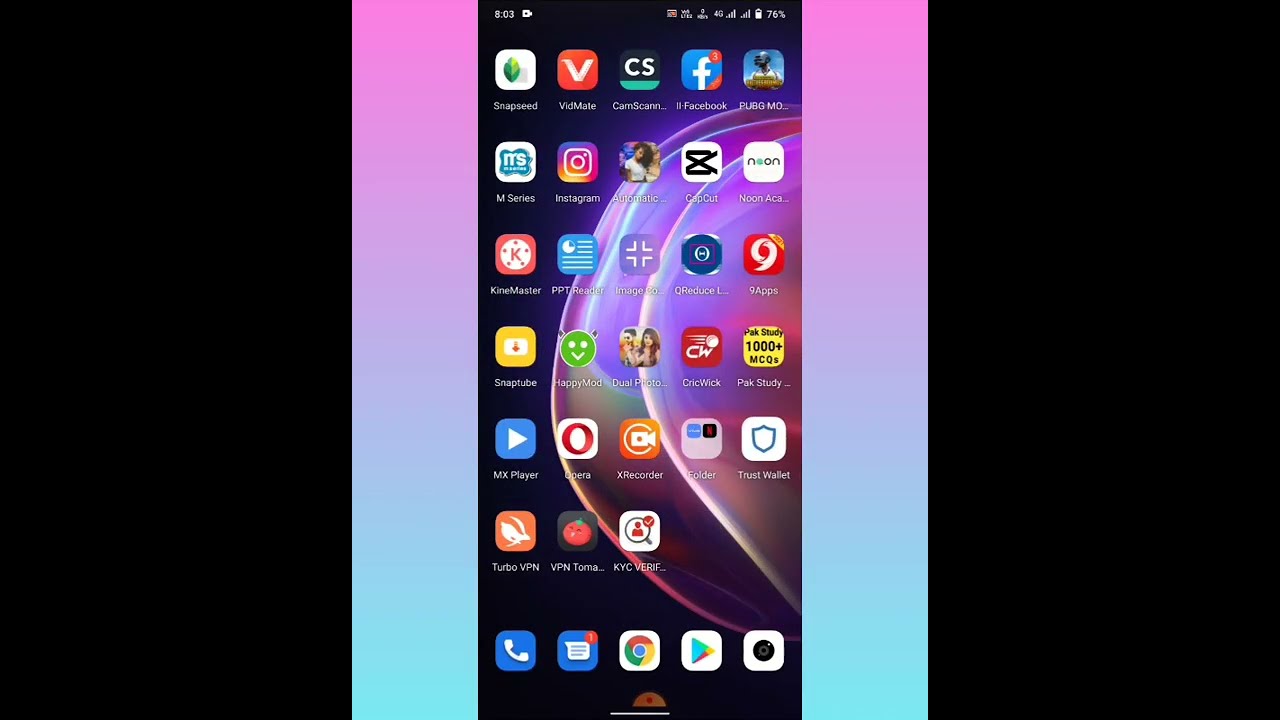This image is a detailed screenshot of a smartphone's home screen, featuring a variety of app icons. The top of the screen displays the time (8:03 AM), battery life at 76%, and several connectivity symbols including 4G signal. The phone's background is a dark theme with a vibrant pink-to-blue gradient bubble in the center, contrasting against the surrounding black bars.

The home screen is structured with seven rows of app icons, although the last row contains only three apps, while the other rows host five apps each. Icon shapes vary, including square, round, and octagonal designs. Prominent apps like Facebook, PUBG, Snapseed, and Instagram are visible among the rows.

At the bottom, the home row features essential apps including the phone call icon in blue, the messaging app with a red notification exclamation mark, Google Chrome, the Play Store, and a camera icon. The sides of the screen have a neon gradient transitioning from bright pink at the top to light neon blue at the bottom, adding a vibrant touch to the phone’s interface.